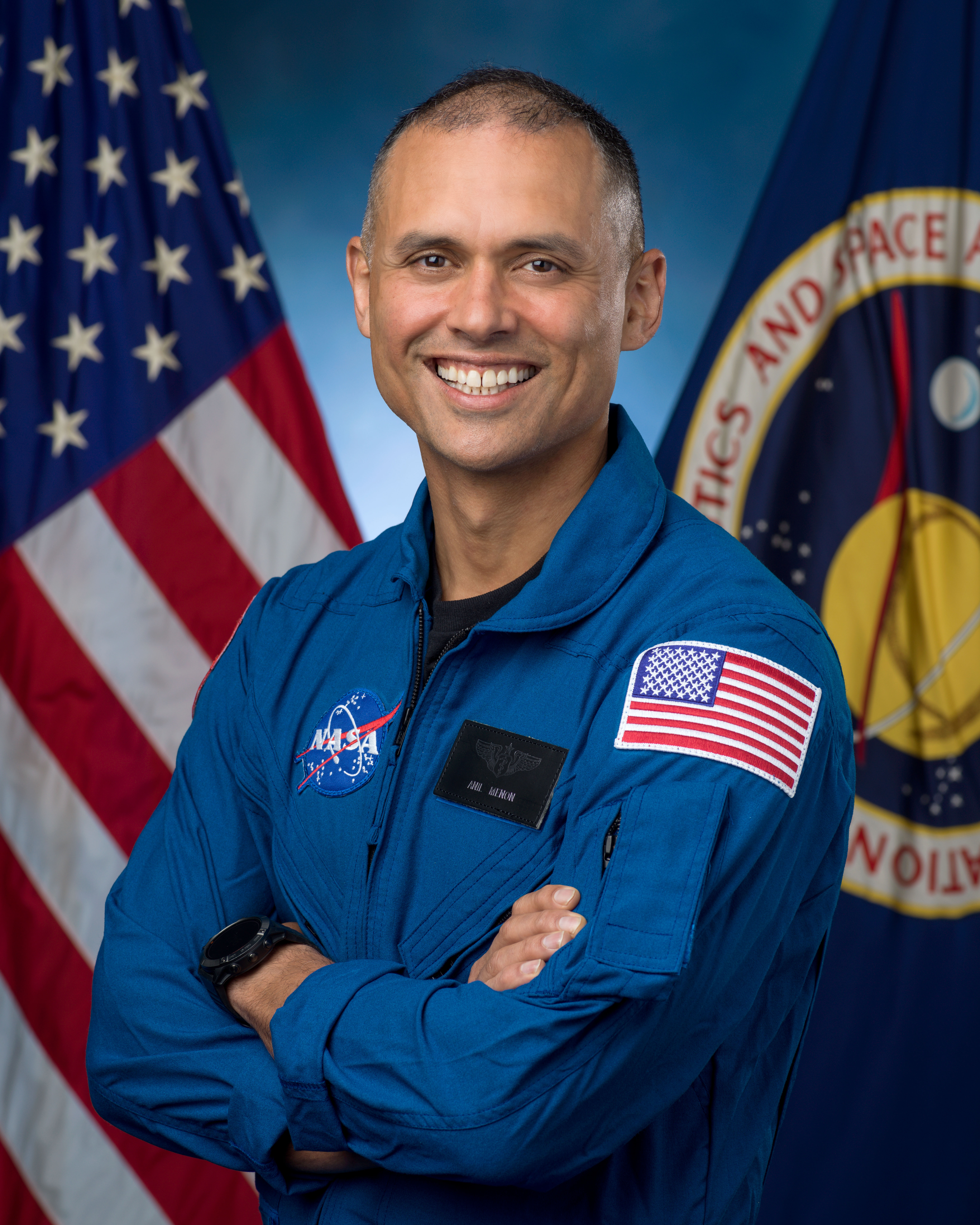This professional photograph features a NASA astronaut standing confidently with a big smile on his face. He is a middle-aged Caucasian man with short, dark hair, lightly balding at the top, and a noticeable tan. Laugh lines around his eyes accentuate his warm smile. He is dressed in a blue NASA flight jacket, which is zipped up. Prominently displayed on his right chest is the iconic circular blue NASA patch with white text, while his left chest bears a black name tag that is not fully legible. His left shoulder is adorned with a distinct American flag patch. He has his arms crossed and is also wearing a black watch on his left wrist. Behind him, the background features the American flag on the left and the NASA flag on the right, which is blue with a white circular emblem that includes the words "National Aeronautics and Space" along with depictions of planets. The image captures the astronaut's professionalism and pride.